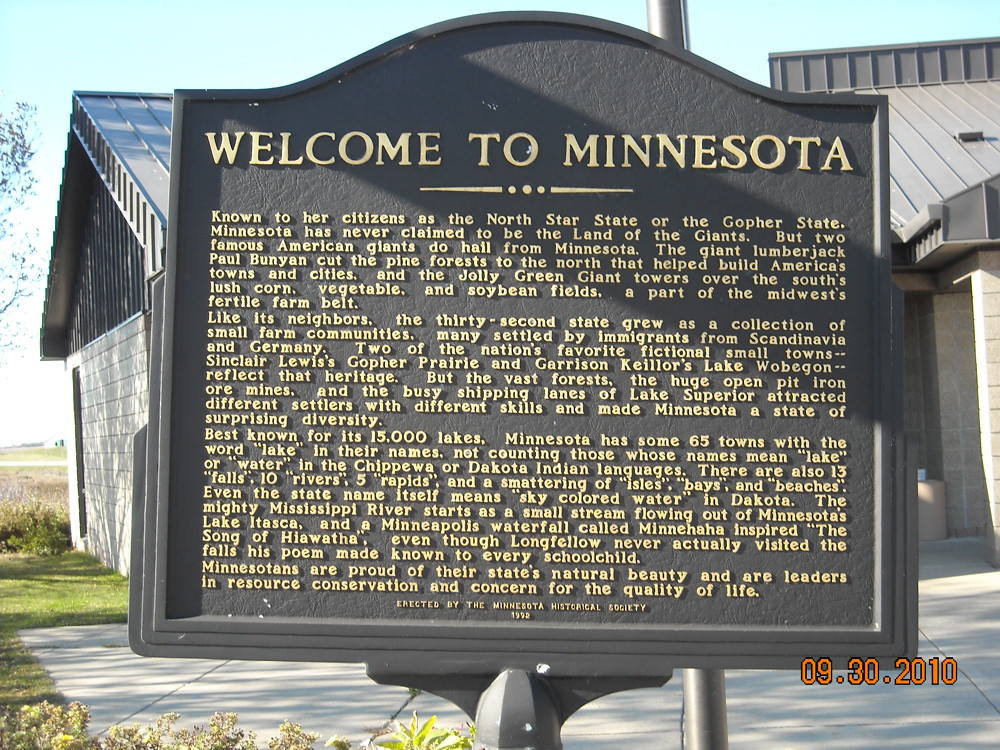This image features a historical marker prominently placed in front of two buildings with metal roofs, one story high and built from white brick, situated in a grassy field. The historical marker, made of metal and black in color with gold text, is the central focus. At the top of the marker, bold text reads, "Welcome to Minnesota." The text highlights Minnesota's nicknames, the North Star State and the Gopher State, and mentions that while the state is not known as the "land of the giants," it is home to two American legends: Paul Bunyan, the giant lumberjack who helped build America's towns and cities by cutting through the northern pine forests, and the jolly green giant who towers over the fertile corn, vegetable, and soybean fields in the south. The marker continues to describe Minnesota's growth from small farm communities into a diverse state with its expansive forests, iron ore mines, and busy shipping lanes on Lake Superior. It mentions the historical importance of towns like Sinclair Lewis's fictional Gopher Prairie and Garrison Keillor's Lake Wobegon, reflecting Minnesota's Scandinavian and German heritage. Further paragraphs emphasize Minnesota's 15,000 lakes, its natural beauty, and the state's leadership in resource conservation and quality of life. The marker was erected by the Minnesota Historical Society, with the date marked as 1992. A timestamp in the lower right of the image indicates the photo was taken on September 30, 2010.